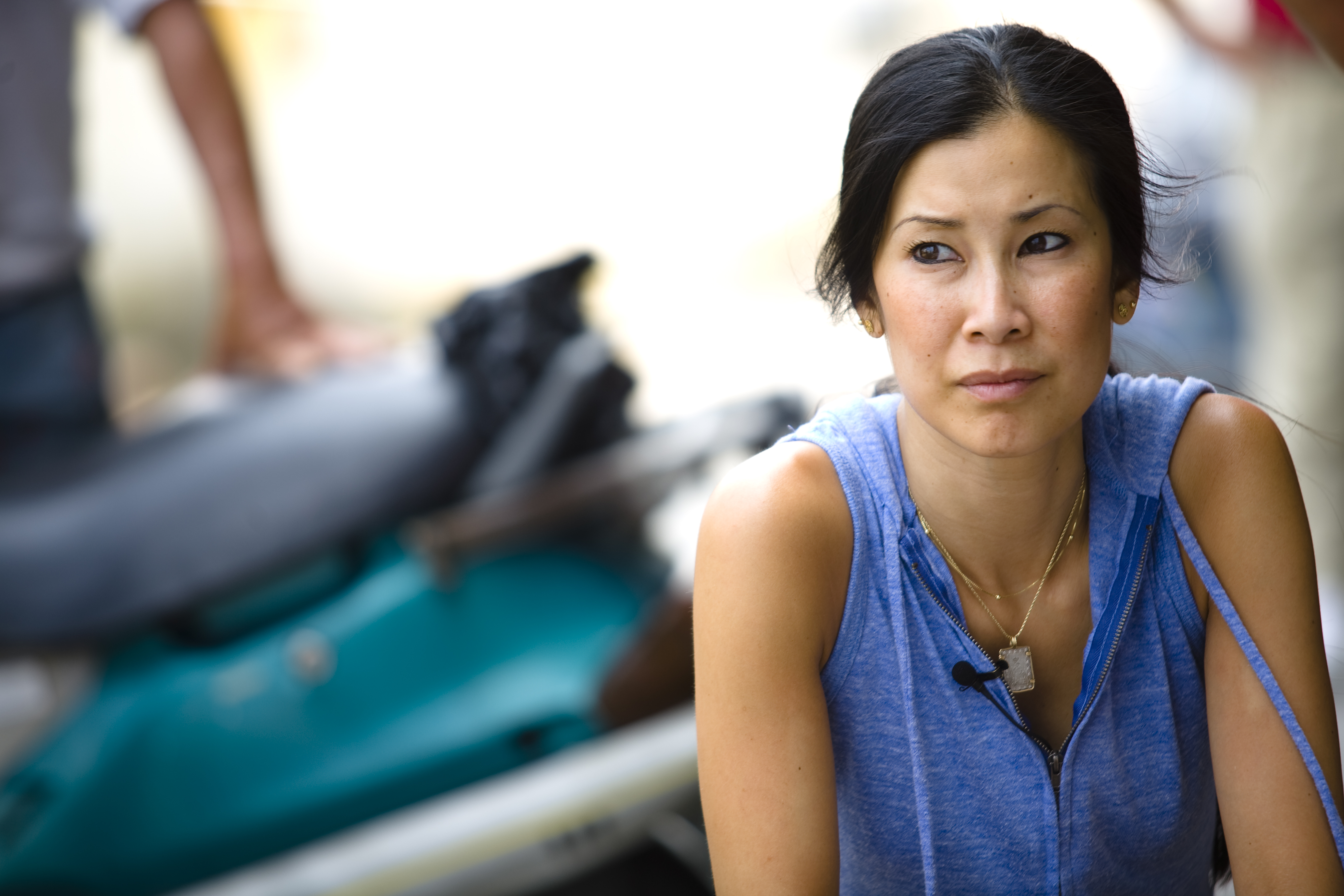The photograph features Lisa Ling, a CNN correspondent, sitting slightly off-center to the right. She is dressed in a light blue, sleeveless jacket with a zipper, giving a glimpse of her gold necklaces underneath, one of which has a rectangular silver pendant. A small black microphone is affixed to her jacket. Lisa, an Asian woman with tan skin, black hair pulled back, and dark eyes, appears to be concerned or worried as she looks off to the left. She wears subtle, ball-type earrings. The background is blurred, but faint details include an outstretched arm in a gray shirt, possible luggage in teal and gray, and sunlight streaming in from the center. Wisps of Lisa's hair suggest an outdoor environment, with the wind gently blowing.